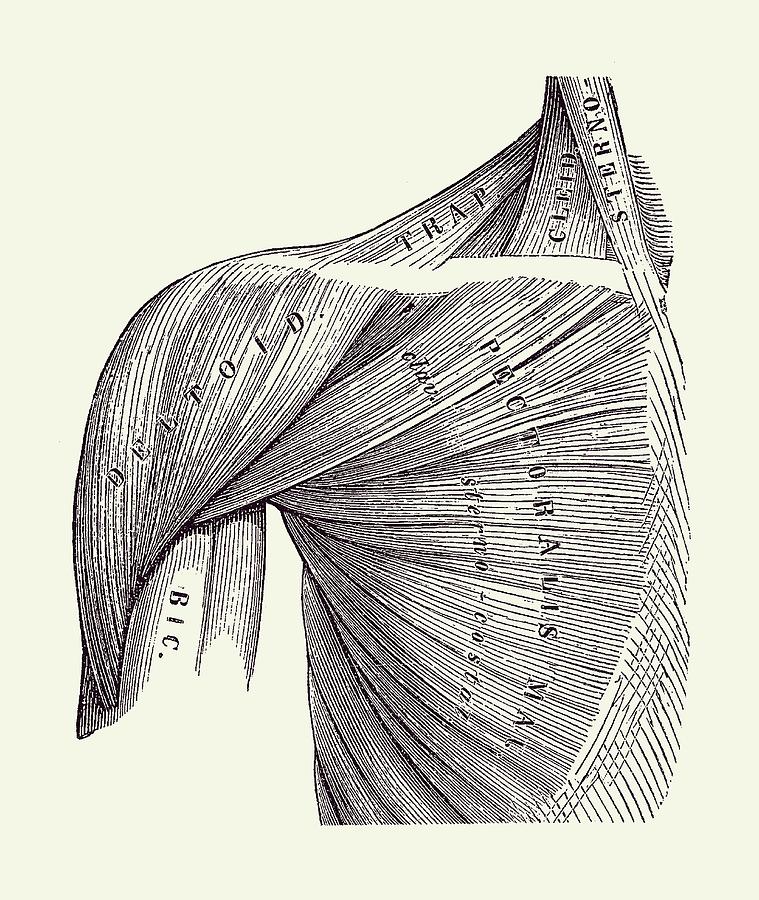The image is a detailed scientific diagram of the human muscular system, specifically focusing on the right shoulder, chest, and neck muscles. The diagram, resembling an intricate pencil etching, features black ink on a solid gray gradient background. It displays the muscles with fine, sketchy, and thinly-lined striations, along with some hatching to indicate depth and articulation. The prominently labeled muscles include the deltoid at the top of the shoulder, the trapezius between the shoulder and neck, the bicep (abbreviated as BIC), pectoralis major (abbreviated as MHA), and several neck muscles including the sternocleidomastoid (abbreviated and partially indecipherable). The overall orientation suggests the figure is facing towards the viewer, with muscles meticulously drawn and labeled to highlight their positions and interrelations within the body.